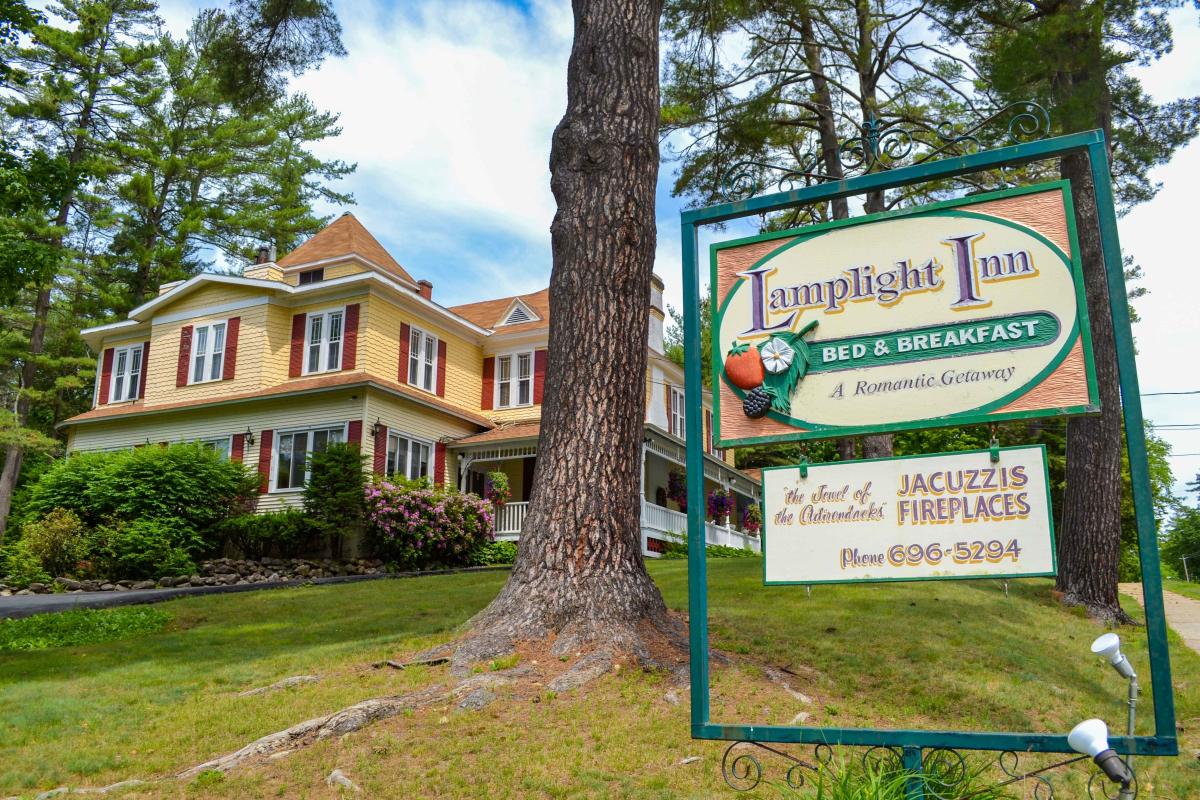The photograph captures a serene scene of the Lamplight Inn Bed-and-Breakfast, nestled on a gentle hill under a bright blue sky adorned with fluffy white clouds. Dominating the image is a large pine tree trunk in the foreground, alongside a prominent, green metal sign with purple writing that reads "Lamplight Inn," and a green banner with white text declaring it as a "Bed and Breakfast". Below, in purple writing, it describes the inn as "A Romantic Getaway," and another white hanging sign promotes amenities such as jacuzzis and fireplaces, listing a phone number (696-5294). The picturesque inn is a two-story beige house featuring windows lined with brown shutters on both levels, a charming wrap-around white porch, and is surrounded by tall, lush trees, green grass, and well-manicured bushes. The roof of the inn is warm orange-brown, complementing the earthy tones of the structure. The scene is completed with a distant road and a glimpse of a path, embodying a peaceful and inviting retreat in the soul of the Adirondacks.